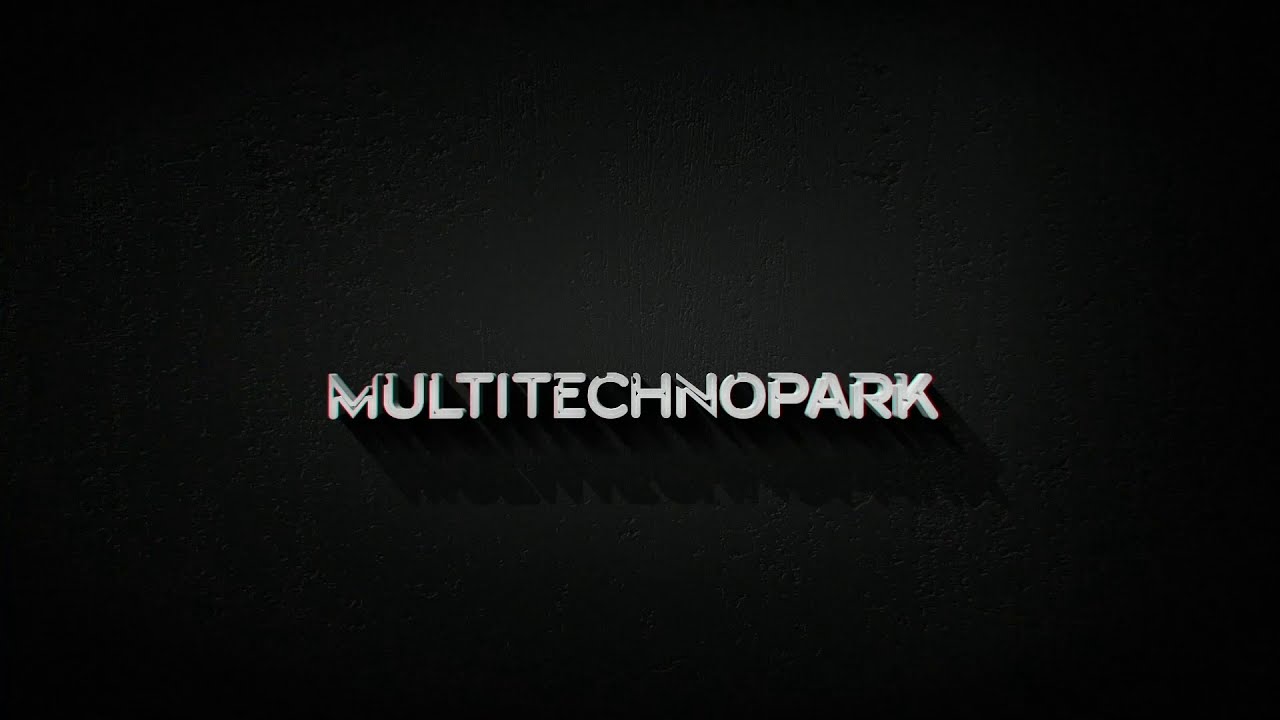The image features a completely black, possibly textured, background with the single word "Multitechnopark" prominently displayed in the center. The text, written in white or off-white with hints of gray, appears to have a shadow effect behind it, adding depth to the lettering. The entire word is capitalized and presented as a single, continuous piece, "MULTITECHNOPARK." Notably, the letter 'M' has a cutout in its center, and similar cutouts are present in the letter 'N,' giving the text a worn, almost "beat-up" appearance. This minimalist composition, devoid of any other objects or text, creates a stark contrast between the striking central word and the vast expanse of empty black space. The arrangement suggests it could be the name of a company, perhaps suited for a website or branding material.